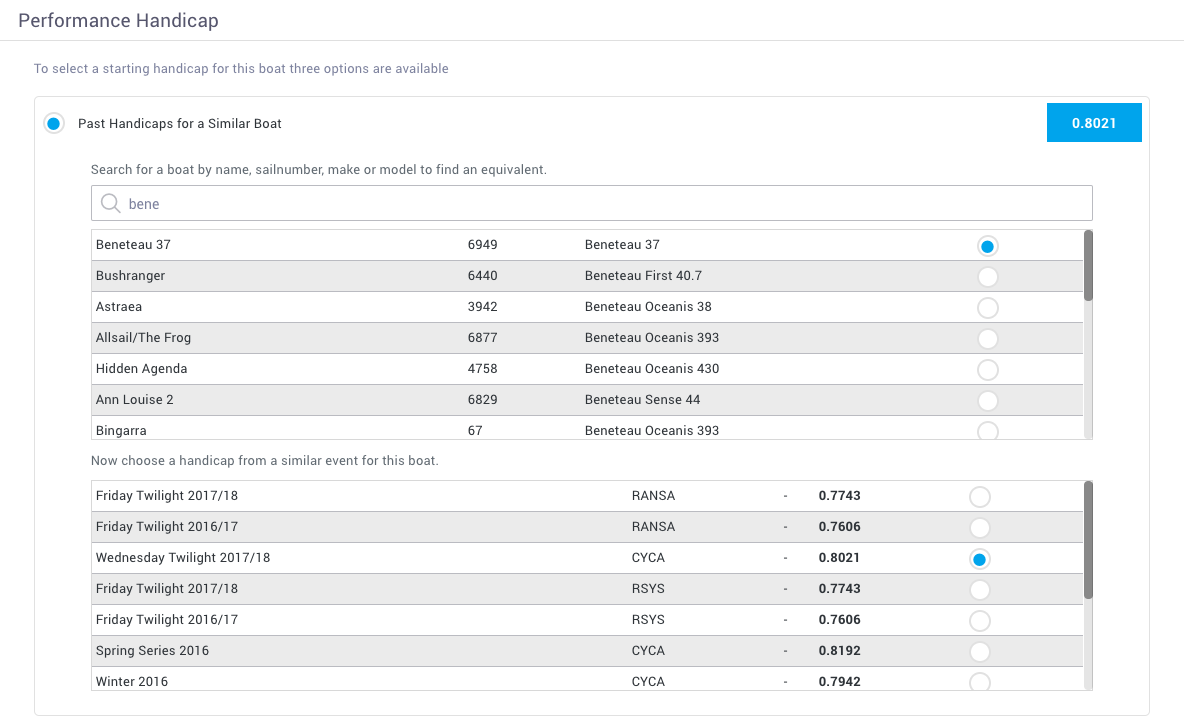The image features a user interface for setting a starting handicap for a boat, presented against a clean white background. There are three options available for selection, each represented by a blue rectangle containing the value "0.8021" on the right side. Additionally, a blue-filled circle is displayed, which indicates the PASS handicaps for a similar boat.

Below these options is a search bar designed for users to find an equivalent boat by name, sail number, make, or model. To the left of the search bar is an icon of a magnifying glass, suggesting its use for searching. The example shown is "BENETEAU 37 6949 Ventenus 37".

Adjacent to the search bar is a blue-shaded dial button, while other sections remain unshaded. Other boats listed include "Bushringer 6440," "First 40.7 Australia 3942," "Oceanis 38," and "ALCEL/SFrog 6877."